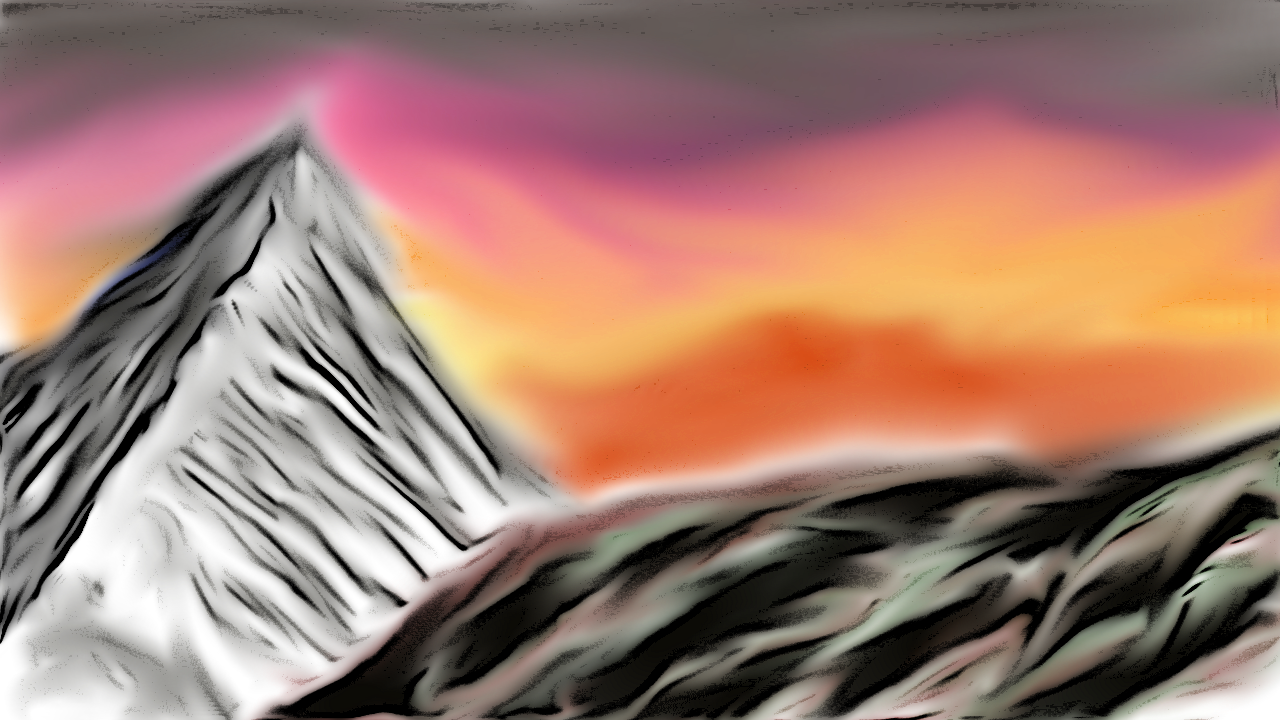This abstract painting captures the essence of a rugged mountain range with vibrant yet textured artistry. The mountains, depicted in shades of white, black, and gray, exhibit a heavily textured, bumpy surface as if countless brush strokes have brought them to life. To the left of the painting, a tall mountain peak stands prominently, while to its right, the incline of another mountain begins to rise. These majestic formations create a valley nestled in the bottom left corner of the piece. Above and around the mountains, a dynamic and colorful sky provides a striking contrast. The sky starts with a warm, orangish hue at the base, transitioning into a thinner band of yellowish-orange, before seamlessly blending into a purple tone that stretches across the upper sections of the mountains. The sky culminates in a dark gray expanse at the very top of the painting. The entire sky appears soft and diffuse, with no defined texture, further emphasizing the mountains' rich, tactile quality.